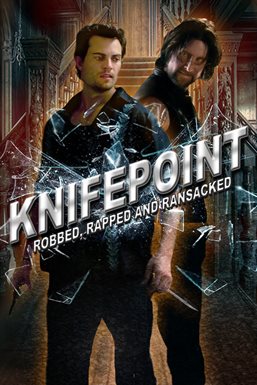The image is a small, vertically oriented rectangle, approximately two inches high and an inch and a half wide. It appears to be an advertisement for a movie or TV show, characterized by a dark, ominous atmosphere. Diagonal white letters, bold and outlined in black, commandingly spell out "KNIFE POINT" across the image, followed by smaller white letters underneath that declare "robbed, raped, and ransacked." 

In the foreground, two men of Caucasian descent stand, seemingly in the midst of a tense moment. The man in the front, dressed in a black leather jacket and jeans, has short dark hair and is gazing off to the right with his hands down by his sides. Behind him, a taller man with longer dark hair, a beard, and a mustache is partially visible, adorned in a black vest. His head is turned over his right shoulder, adding to the sense of unease.

The background hints at a dilapidated, possibly haunted house, complete with an eerie staircase that enhances the unsettling mood. Further details include broken glass scattered around, contributing to a scene that feels chaotic and dangerous. The overall design, coupled with spiderweb-like graphic elements, induces a sense of dread and suspense typical of horror or thriller genres.